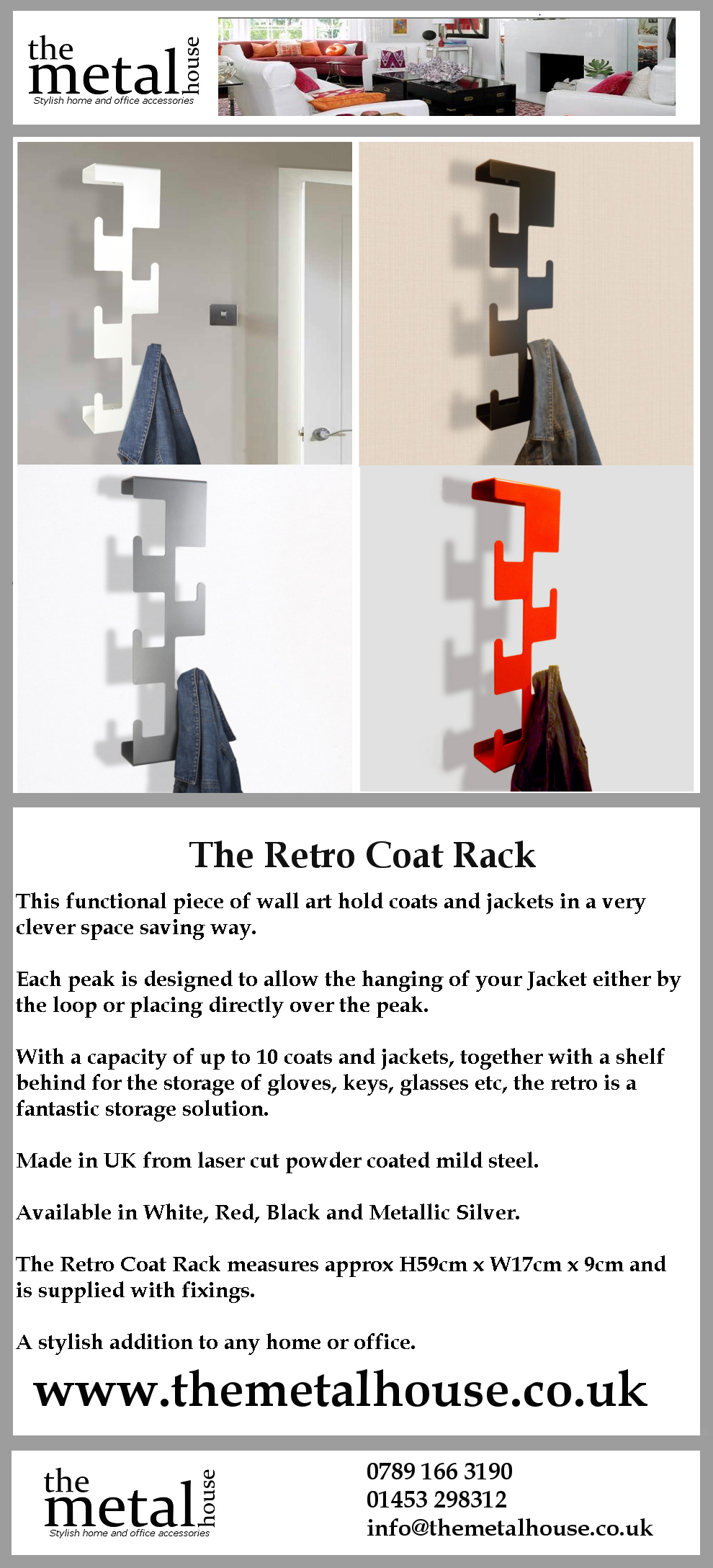The advertisement features a product known as "The Retro Coat Rack" by The Metal House. The visual layout includes a prominent horizontal banner at the top displaying "The Metal House" in white text over a small, narrow image of a cozy interior, highlighting furniture such as a white couch, a red pillow, an orange pillow, and a white-covered fireplace.

Beneath this banner, there are four different photos of The Retro Coat Rack displayed in various colors: black, red, white, and metallic silver. Each image shows the coat rack installed on a wall, with a single coat hung on one of its lower pegs. In each photo, adjacent details include elements like a white door, light brown and off-colored walls, other clothing hangers, and shirts in various colors, emphasizing the contrast and compatibility of the coats with the racks.

Below these images, a white field with black text contains the product's detailed description. It reads: "The Retro Coat Rack, The Functional Piece of Wall Art. This functional piece of wall art holds coats and jackets in a very clever, space-saving way. Each peak is designed to allow the hanging of your jacket either by the loop or by placing directly over the peak. With a capacity of up to 10 coats and jackets, together with a shelf behind for storing gloves, keys, glasses, etc., The Retro is a fantastic storage solution. Made in the UK from laser-cut, powder-coated mild steel, available in white, red, black, and metallic silver. The Retro Coat Rack measures approximately 59 cm by 17 cm by 9 cm and is supplied with fixings." Additionally, the product is touted as a stylish addition to any home or office.

At the bottom of the advertisement, contact information is provided: the website www.themetalhouse.uk and the phone number 0789-166-3190.